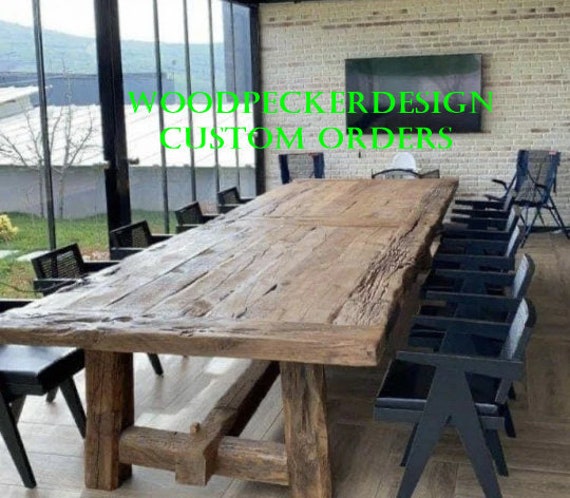The photograph, an indoor scene with a focus on a long, rustic wooden table crafted from rough-hewn planks, captures the essence of design and functionality in a modern meeting space. Central to the image, the table is surrounded by black chairs, most of which are matching wooden seats while a distinct, folding black chair stands out mid-right. The background features a light-colored brick wall with scattered red bricks and a large flat-screen TV mounted on it. Floor-to-ceiling windows on the left provide a clear view of a small grassy area with concrete steps, leading to a white shed-like building, with hills or mountains visible in the distance. The text "woodpecker design custom orders" in bold lime green letters adorns the top center of the image, adding a promotional touch. The setting combines modern aesthetics with a touch of natural ruggedness, further emphasized by the light-colored wood plank flooring.